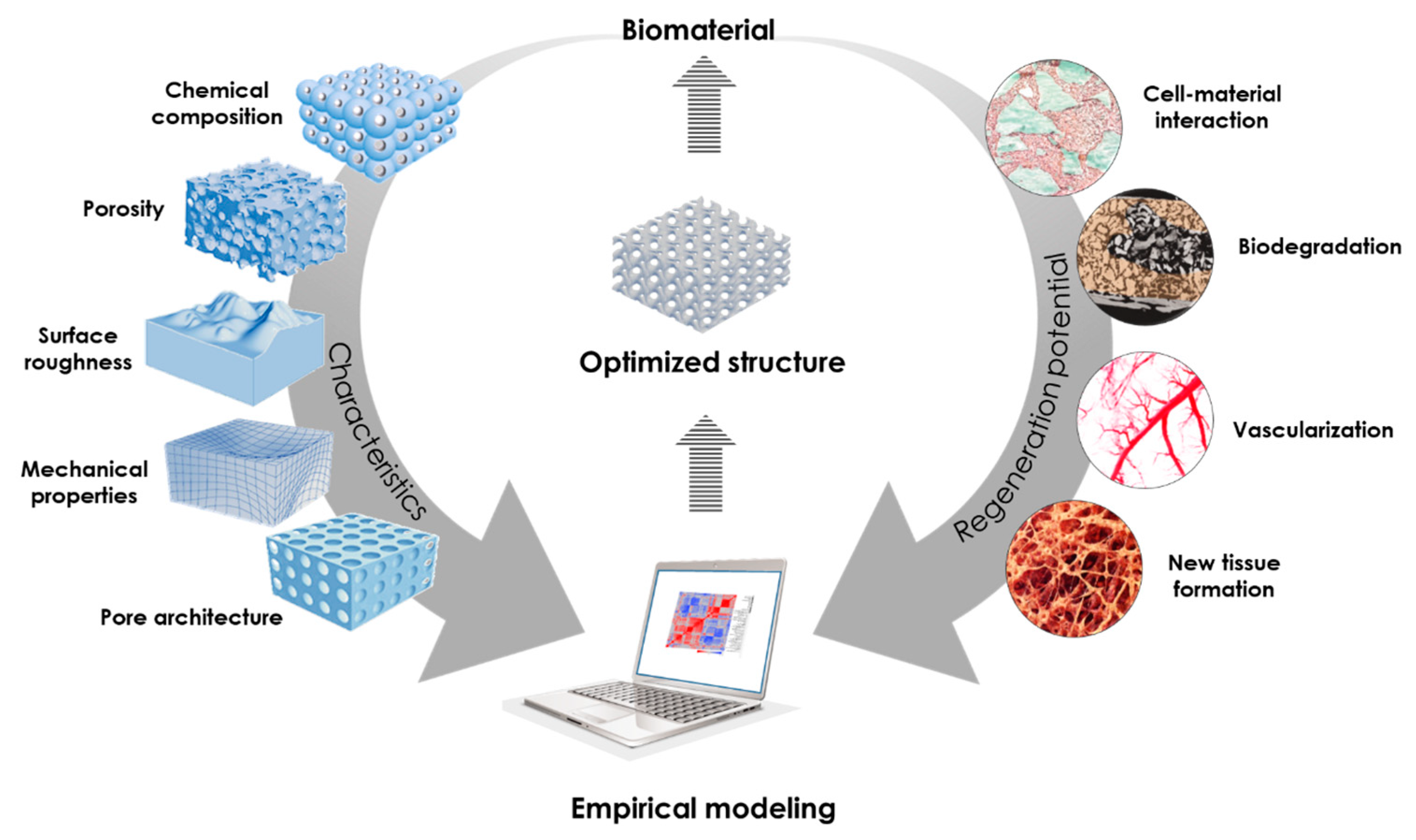The scientific graphic illustrates the holistic process of biomaterial optimization and empirical modeling on a white background. At the core is a labeled "Biomaterial." Starting from the biomaterial, two large gray arrows form a circular pathway. The arrow on the left side is labeled "Characteristics" and points downward, presenting five distinct characteristics: "Chemical Composition," "Porosity," "Surface Roughness," "Mechanical Properties," and "Pore Architecture," each depicted with blue-textured cubes. On the right side, the arrow is labeled "Regeneration Potential," showcasing four stages: "Cell Material Interaction" (illustrated with close-up images in blue and light pink), "Biodegradation," "Vascularization" (featuring images of vascular veins), and "New Tissue Formation."

Both arrows converge towards a laptop at the bottom labeled "Empirical Modeling." An additional arrow points up from the laptop to an object labeled "Optimized Structure," connecting back to the "Biomaterial" at the top, depicting the cyclical process of refining and enhancing biomaterials. This detailed diagram, complete with images and descriptive labels, encapsulates the stages and considerations integral to developing advanced biomaterials and their applications in tissue regeneration.